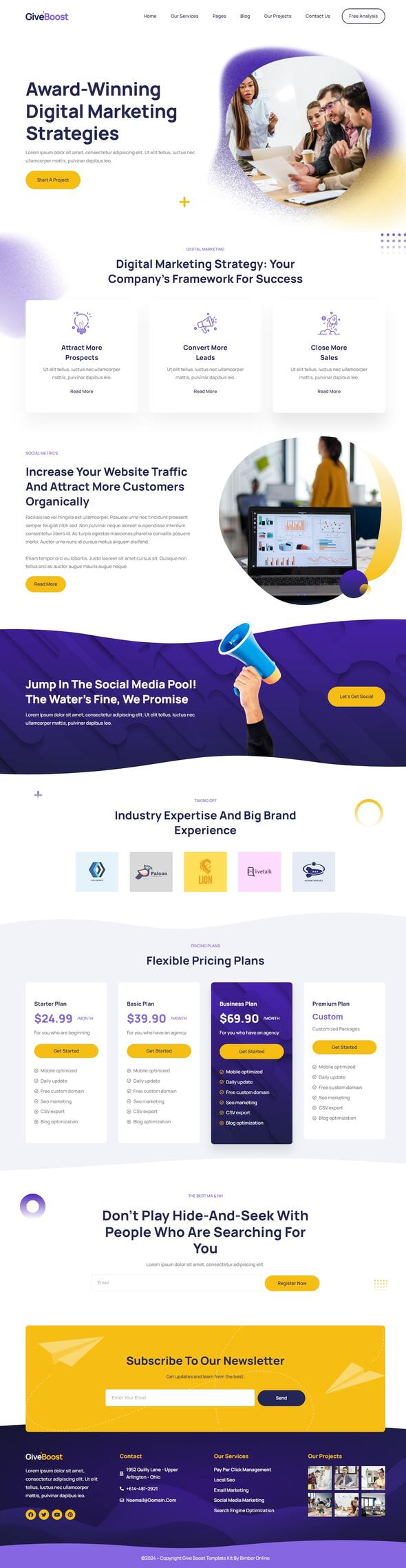This image depicts the homepage of the award-winning digital marketing agency, Give Boost. The headline boldly introduces their expertise in creating effective digital marketing strategies tailored to ensure your company's success. Key features spotlighted include enhancing prospect attraction, increasing lead conversion, driving more sales, boosting website traffic, and expanding customer acquisition.

A playful call-to-action encourages businesses to engage with social media, humorously assuring, “Jump in the social media pool, the water’s fine, we promise.” The organization prides itself on its industry expertise and experience with major brands. Various flexible pricing plans are highlighted: a Starter Plan at $24.99 per month, a mid-tier plan at $39.99 for three months (or potentially two months), a Business Plan at $69.99, and a customizable package tailored to specific business needs.

The site also emphasizes the importance of visibility with a catchy phrase: "Don’t play hide and seek with people who are searching for you," encouraging visitors to subscribe to their newsletter for the latest updates.

At the bottom, the footer provides the company's contact information, indicating their location in Upper Arlington, Ohio. It also details the range of services offered, including Pay Per Click Management, Local SEO, Email Marketing, Social Media Marketing, and Search Engine Optimization. The comprehensive and well-structured presentation aims to convey both professionalism and accessibility.